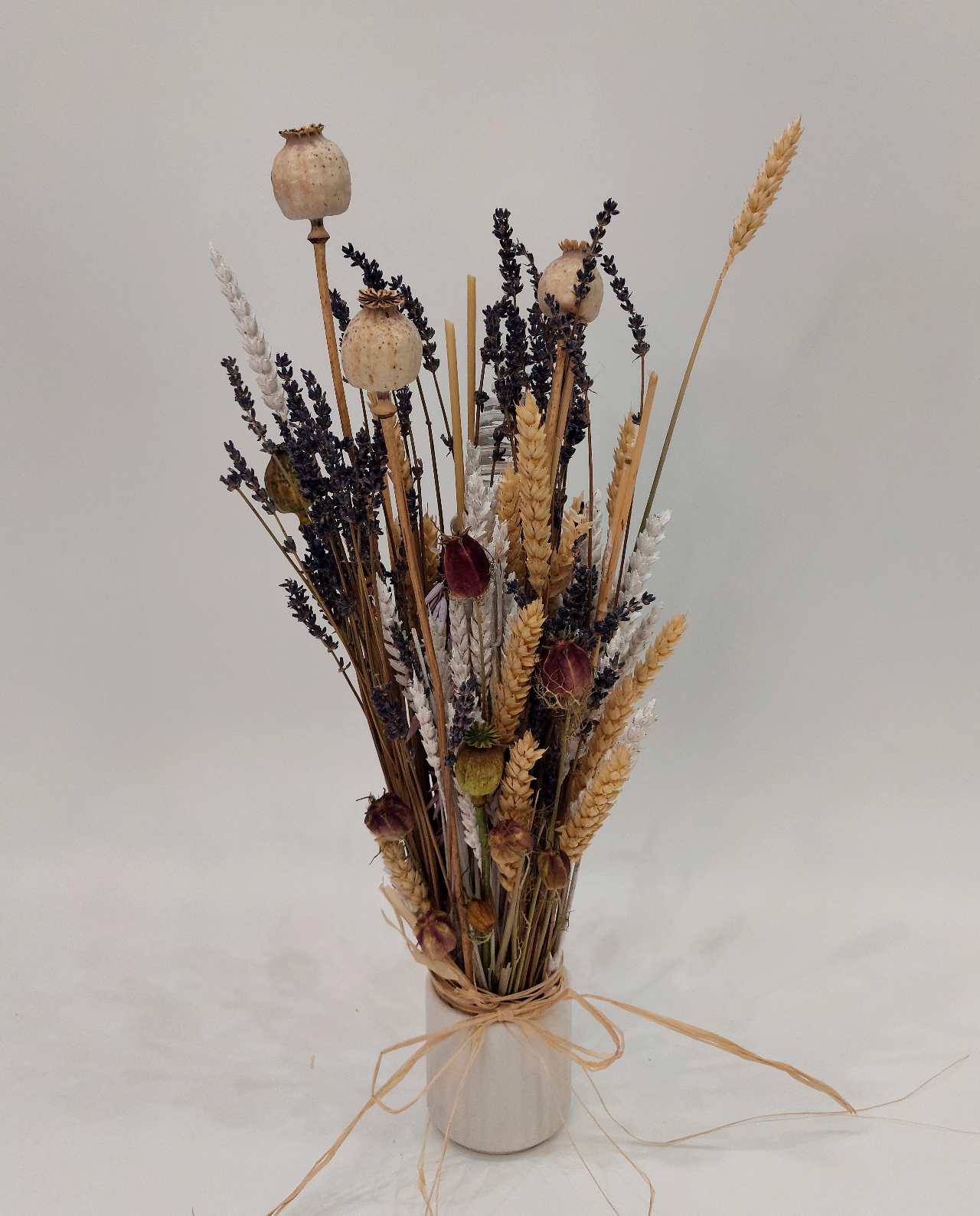This is a detailed photograph of a professionally arranged floral bouquet set against a pure white background. The arrangement is placed in a small, white jar-shaped vase adorned with a light brown, straw-textured ribbon tied around the top. The bouquet features a diverse collection of elements, including stalks of wheat and dried poppy pods on long, pale brown stems. The vibrant assortment of colors includes white, dark purple, dark pink, yellow, and hints of green. Some of the stalks appear more leafy, though they are not leaves. The preserved poppy pods, along with various bulbs, wheat berries, and potentially wilted flowers, create a harmonious blend that exudes an autumnal or wintry feel. This carefully curated arrangement, which occupies most of the image, suggests a professional touch suitable for use in a website, magazine, or as an advertisement.